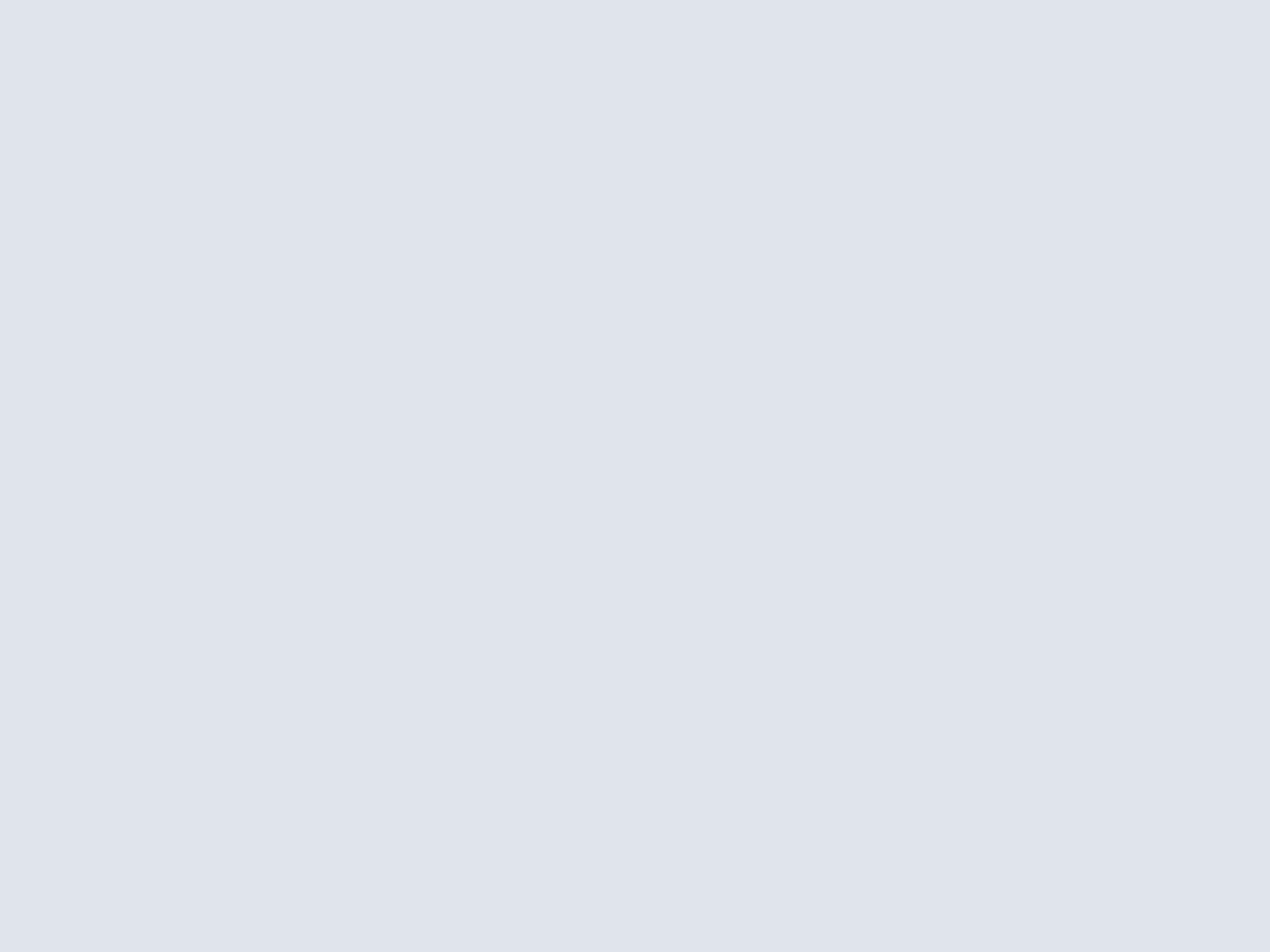An image entirely devoid of any distinguishable features or elements, presenting a uniform, uninterrupted expanse of gray. The absence of objects, text, or any discernible details creates a stark, minimalist visual experience characterized by its complete emptiness and simplicity.